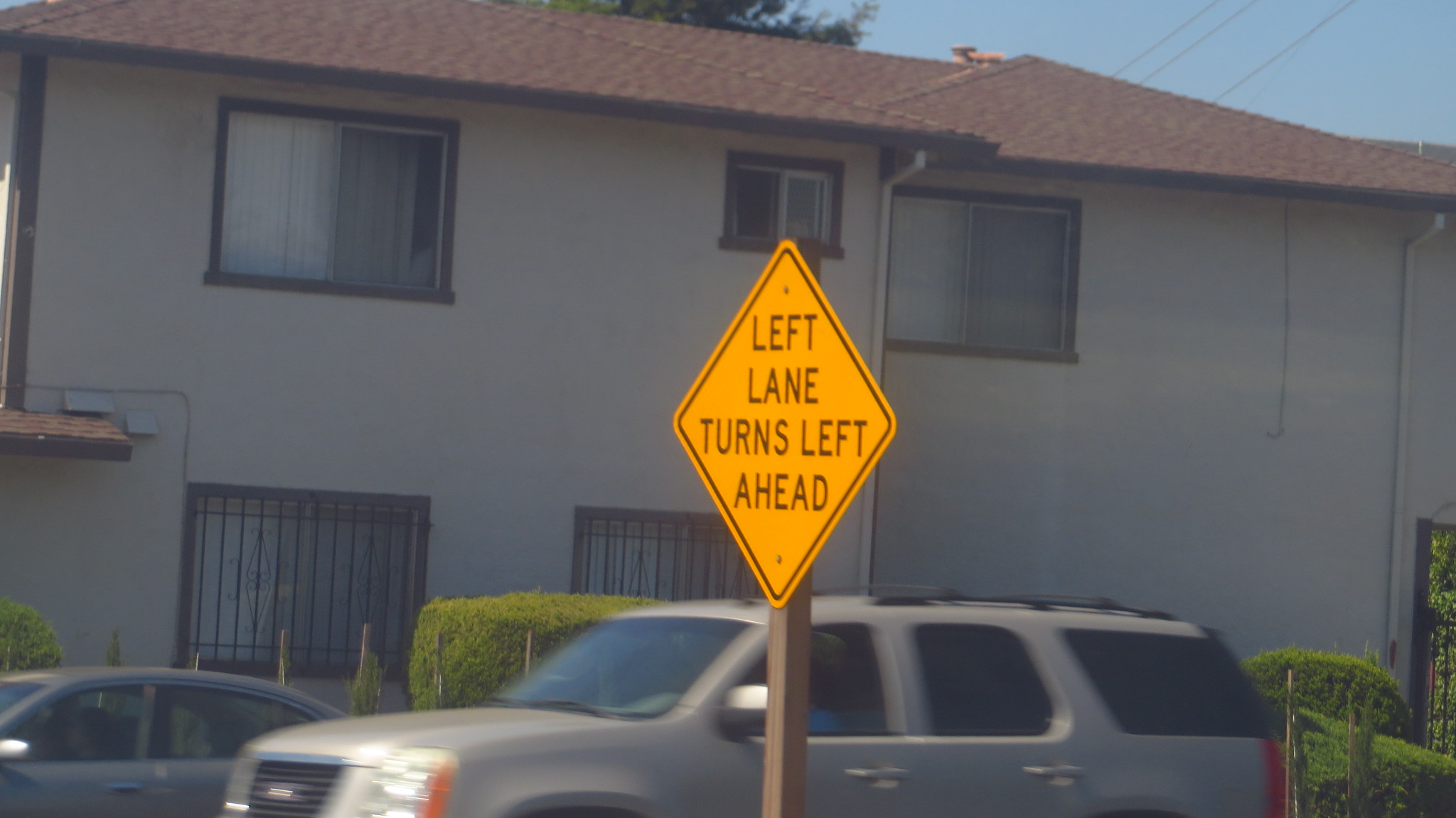In this photograph, we see a prominently positioned diamond-shaped street sign with a yellow background and black trim. The sign, which states "Left Lane Turns Left Ahead" in black text, is attached to a post beside a road. Two vehicles are passing by the sign: a light brown or grayish SUV in the foreground and a gray compact sedan partially visible. Behind these vehicles, there's a large, two-story building that resembles an apartment complex. The building has a light whitish cream or gray exterior with black or brown trim around the windows, which are adorned with vertical blinds inside and vertically placed metal bars on the lower windows. The roof is covered in reddish-brown tiles, and above it, there are telephone or electrical wires and a glimpse of trees and blue sky. The scene also includes some hedges and various wires and gutters clinging to the building’s facade.